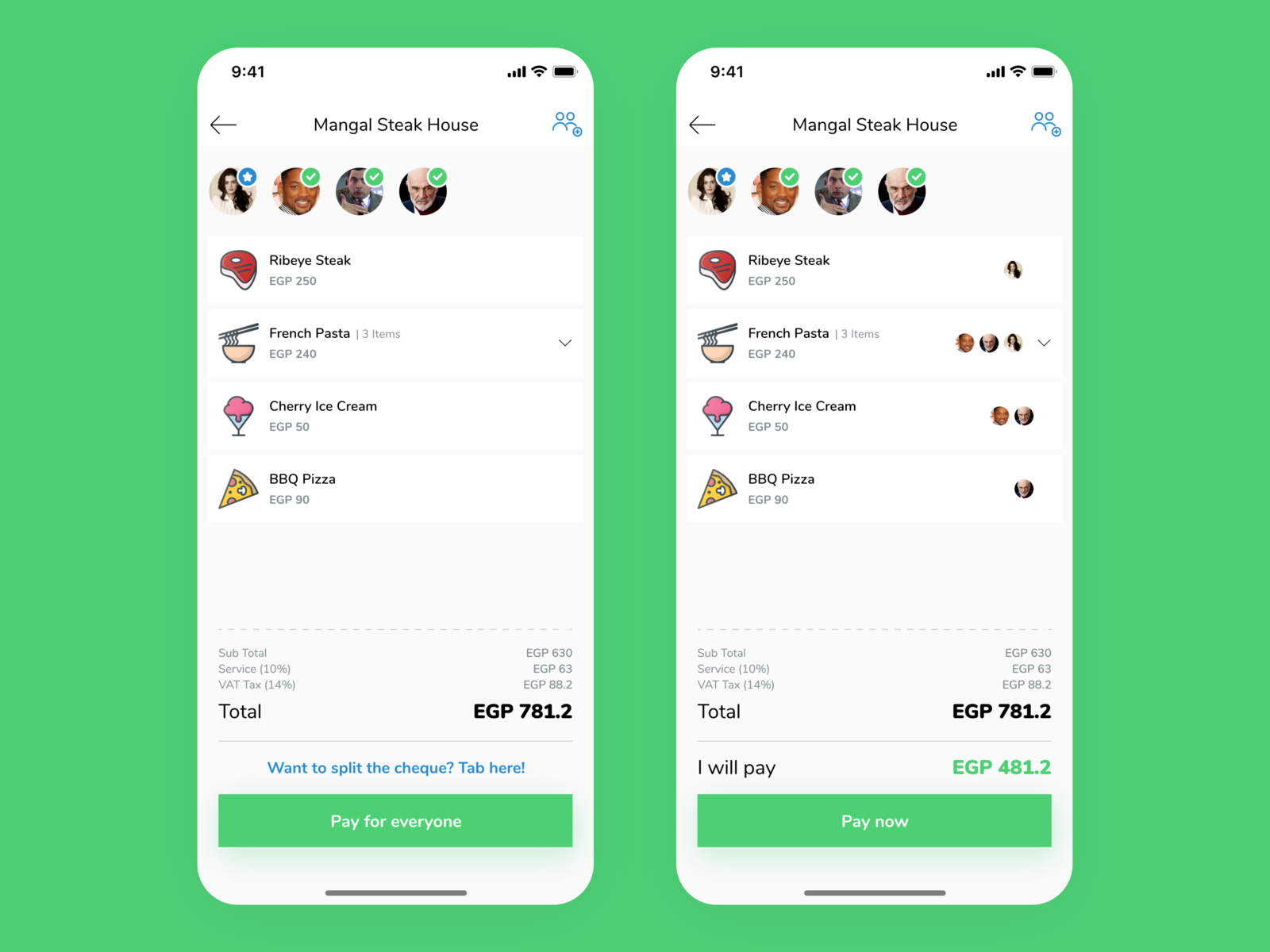Two smartphones are placed side-by-side against a green background. The screen on the left displays a transaction from "Mangal Steakhouse" with a total amount of EGP 781.2. It includes a prompt at the bottom inviting the user to "split the check" by tapping for options to "pay for everyone." The screen on the right shows a similar transaction for "Mangal Steakhouse" but highlights an option at the bottom stating, "I will pay 481.2," with a "pay now" button.